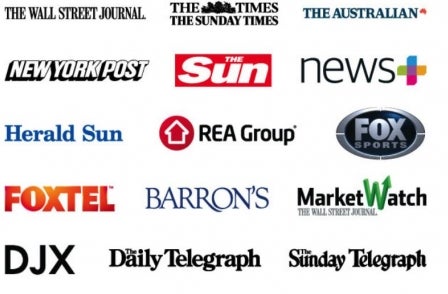The image features a collage of various company names and logos arranged against a solid white background. 

- **Top Row (from left to right):**
  - The Wall Street Journal (rendered in classic black text)
  - The Times
  - The Sunday Times (both in traditional serif fonts)
  - The Australian (placed in the upper right corner)

- **Second Row (from left to right):**
  - New York Post (depicted in its recognizable block letters with shadow)
  - The Sun
  - News+ (stylized as one word: "NewsPlus")

- **Third Row (from left to right):**
  - Herald Sun (in blue text)
  - The Re-group (featuring a red circle with a white arrow inside it)
  - Fox Sports (displayed in a logo shaped like a football, colored silver and blue)

- **Fourth Row (from left to right):**
  - Foxtel (in bold orange block text)
  - Barron's
  - MarketWatch
  - The Wall Street Journal again

- **Bottom Row (from left to right):**
  - DJX
  - The Daily Telegraph
  - The Sunday Telegraph

Each logo and name is distinctly styled, providing a comprehensive visual representation of various media and news entities.